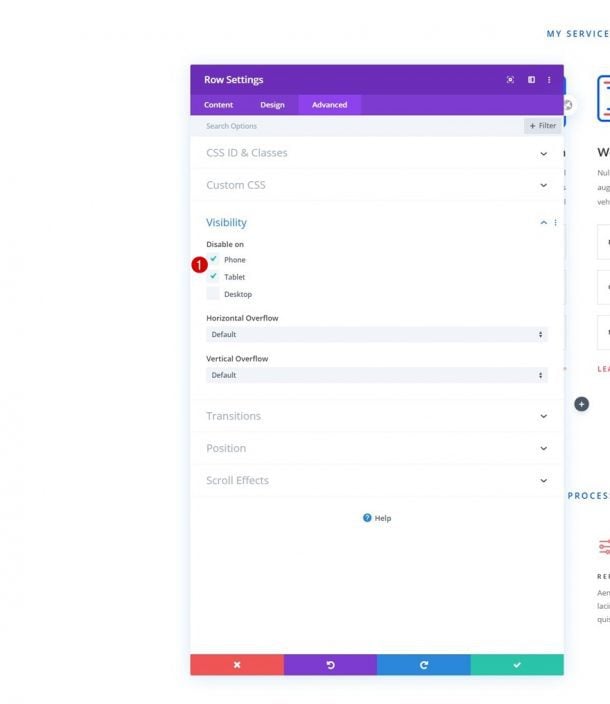This is a detailed screenshot of a mobile app interface that resembles a Windows 8 application. The top of the screen features a distinct purple bar with white text that reads "Row Settings." Below this header are three tabs labeled "Content," "Design," and "Advanced," with the "Advanced" tab currently highlighted.

In the main section of the screen, under a gray bar that reads "Search Options," is a filter button positioned to the right. Underneath this section, there are multiple drop-down menus. The first is labeled "CSS ID and Classes," followed by another labeled "CSS Custom."

The "Visibility" drop-down menu below that is expanded, displaying options for device visibility. The selections indicate that the options for "Phone" and "Tablet" have been marked with checkmarks and have a red circle with the number one next to them, signifying active selection. The "Desktop" option, however, remains unchecked.

Further down, the settings for "Horizontal Overflow" and "Vertical Overflow" are both set to default values. Following these, there are drop-down menus for "Transitions," "Position," and "Scroll Effect."

At the very bottom of the screen, navigation controls are displayed, including buttons for exit, go back, go forward, and a check button for confirmation.